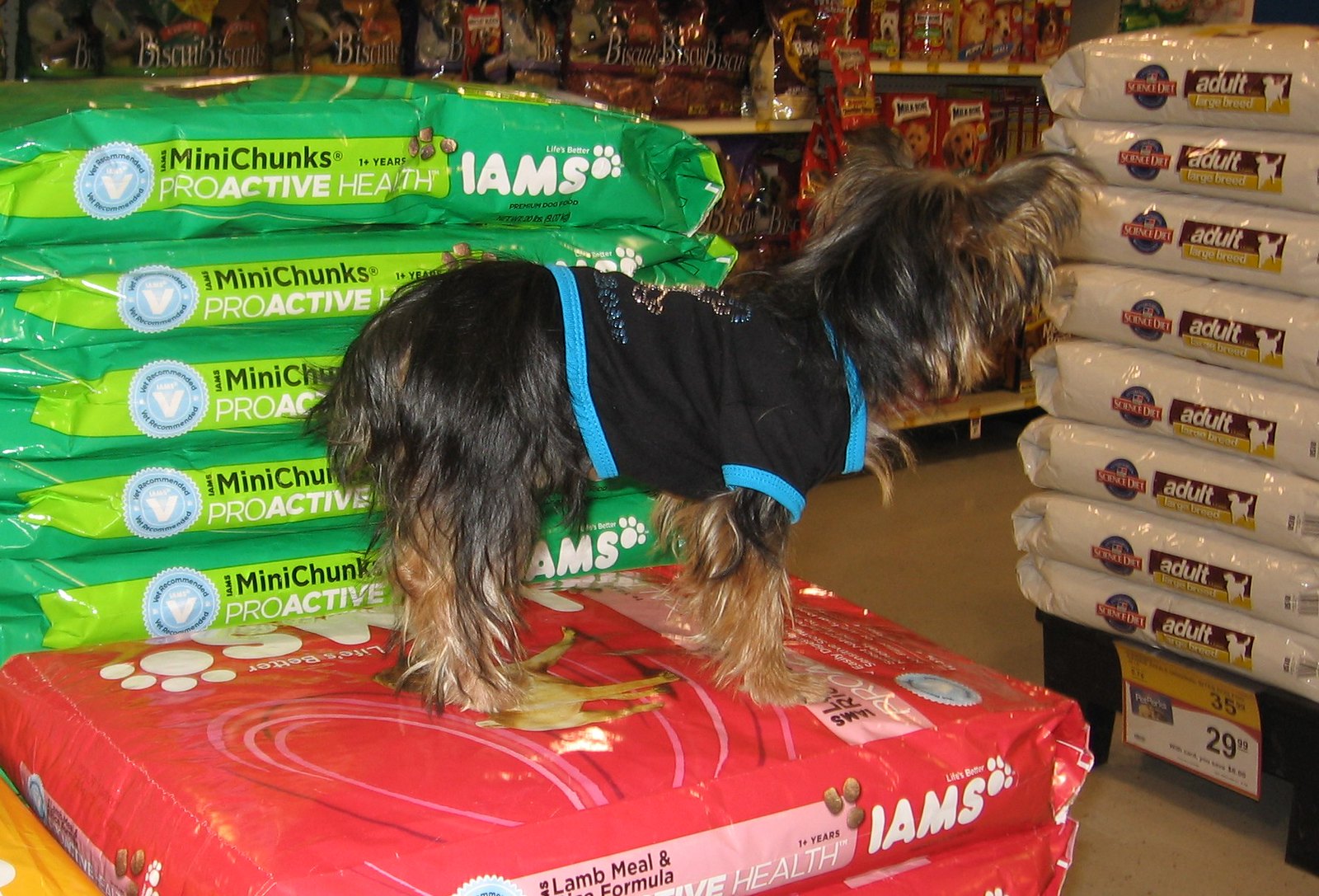This indoor photograph depicts a small brown dog dressed in a black jacket with blue trim. The dog is perched atop a red IAMS bag of dog food. Surrounding the dog are five stacks of green IAMS Mini Chunks Active dog food bags, and prominently featured text includes "Proactive Health" and "Lamb Meal & Rice Formula." The dog's gaze is directed towards a pallet on which eight more bags of dog food are mounted. In the background, shelves stocked with various pet food items, including red bags, are visible. The flooring of the setting is dark brown, adding a contrasting backdrop to the colorful assortment of pet products in what appears to be a pet supply store.